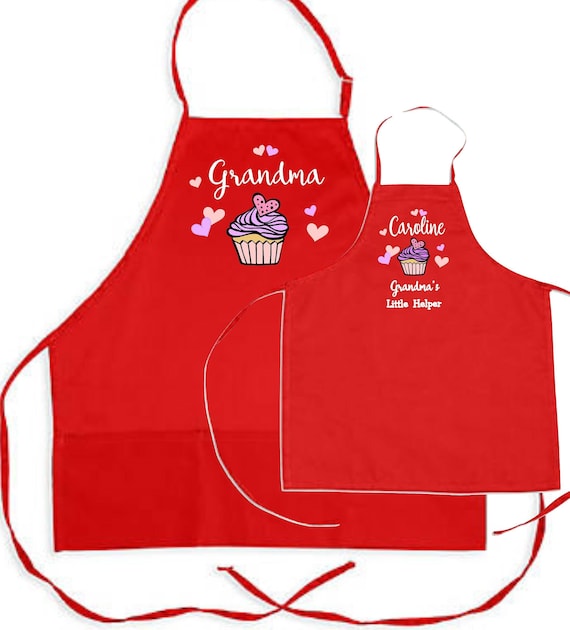This vibrant image showcases two matching aprons set against a solid white background, perfect for a sale listing on a customization website like Etsy. The larger apron, designed for an adult, is entirely red with long straps and a neck loop. It features the word "Grandma" elegantly printed in white letters at the top, with charming pink and purple hearts adorning both sides, and a cute purple cupcake with a decorative pink heart on top below the text.

Overlaying the adult apron is a smaller, child-sized apron in the same vivid red color. It mirrors the design of its larger counterpart, with "Caroline, Grandma's Little Helper" inscribed in white letters. Like the adult apron, it is decorated with pink and purple hearts and the same whimsical cupcake graphic. The clear and bright natural lighting enhances the vividness of the red aprons and the detailing of the designs, making the entire setting visually appealing and easy to view.